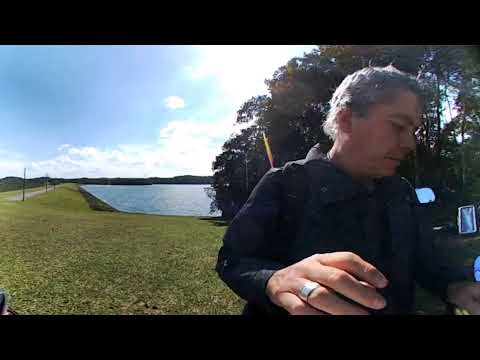In this outdoor photograph taken on a sunny day, a middle-aged man with short-cropped gray hair occupies the right side of the frame. Clad mostly in shadow, his face and body are silhouetted, making details hard to discern. Notably, his right hand is illuminated by sunlight, revealing a silver band on his ring finger. The man gazes downward and slightly to his left, his left hand barely visible in the darkness. Above this hand, three vertical, luminous objects add a hint of mystery to the scene. The background behind him features a stand of trees with the bright, low-horizon sun shining from behind, casting a radiant glow over the central clouds. Dominating the left half of the photograph is a picturesque landscape of low-cut green grass leading to a serene lake or reservoir. The water, a reflective blue, stretches to the horizon where a thin strip of land and a trail with posts add depth to the scene. Silvery-white clouds adorn the blue sky, illuminated by the sunlight. The overall setting appears to be a park or natural area, most likely during spring or summer.